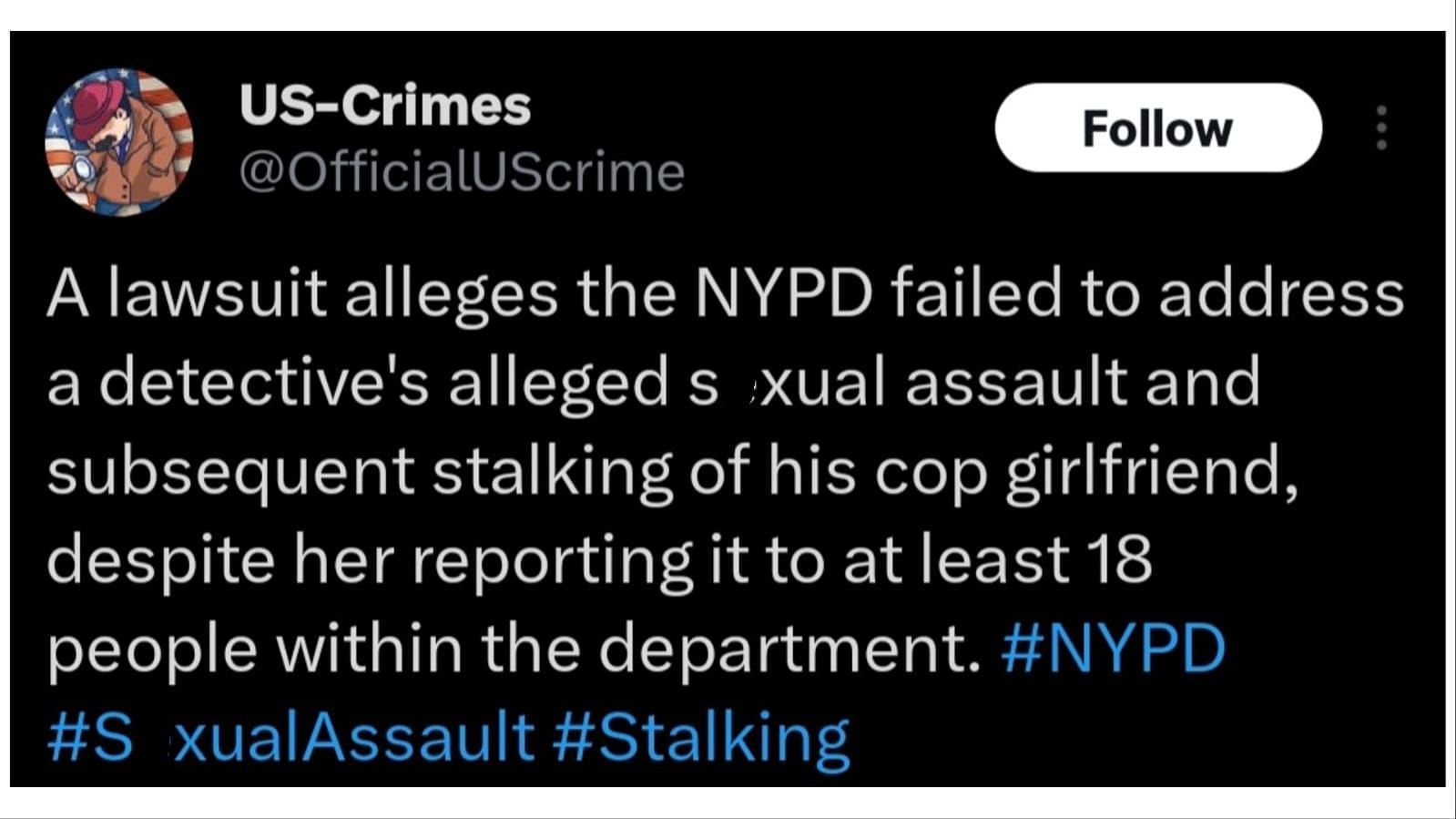This image, originating from a social media post, features a predominantly black background with the heading "U.S. Times" at the top. Centrally featured is a cartoon illustration of a man standing before the American flag. In the top right-hand corner, there is a 'Follow' button accompanied by three vertically aligned gray dots, indicating additional options. 

White text on the black backdrop reads: "A lawsuit alleges the NYPD failed to address a detective's alleged sexual assault and subsequent stalking of his cop girlfriend, despite her reporting it to at least 18 people within the department." Noteworthy hashtags in blue include #NYPD, #sexualassault, and #stalking. However, the text "sexual assault" and the corresponding hashtag have been obscured with black marker ink, highlighting an attempt at censorship or redaction.